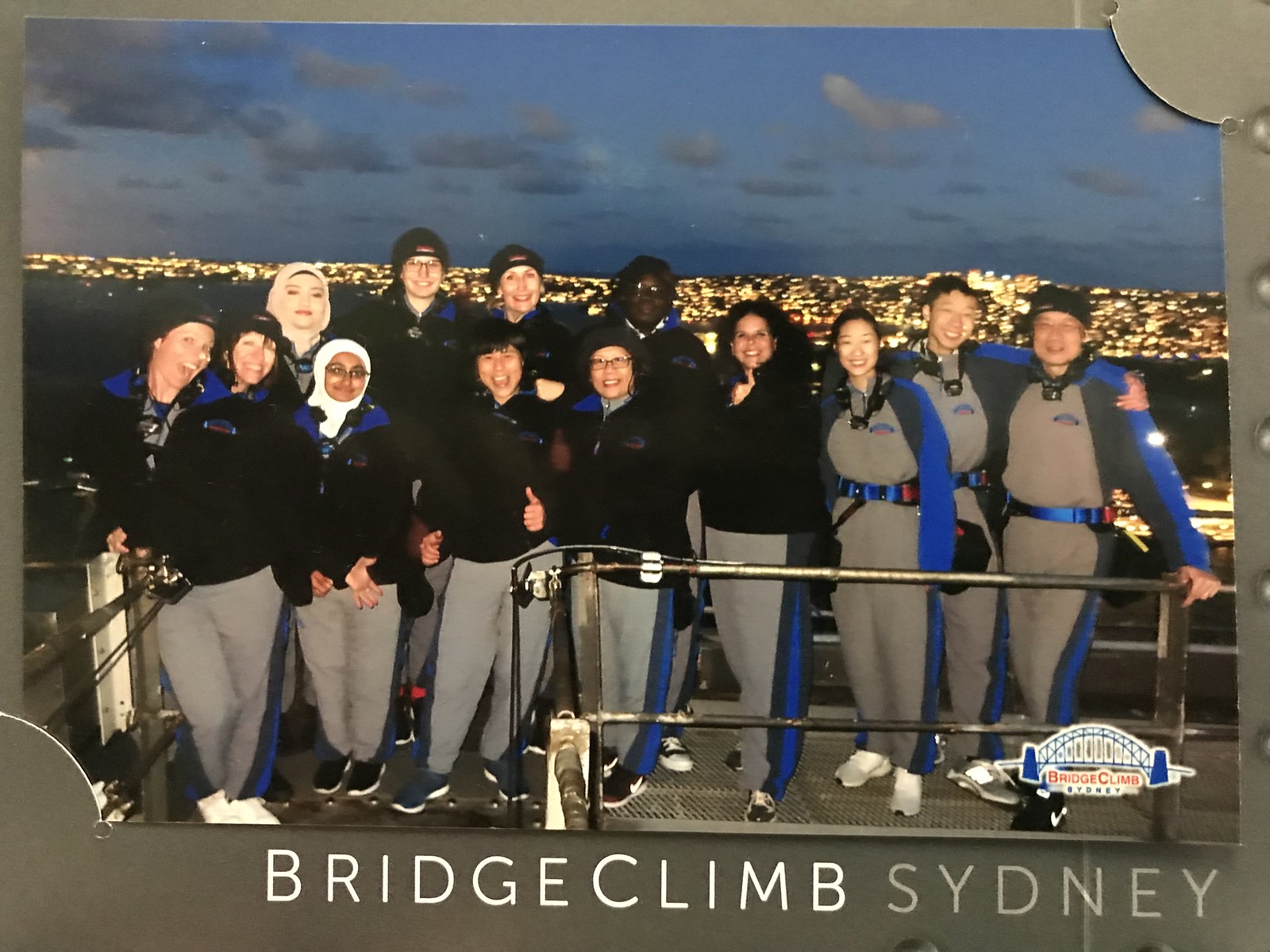This photograph captures a postcard-worthy moment featuring a diverse group of 13 people standing on a platform, decked out in matching bridge-climbing uniforms. The uniforms are gray jumpsuits with distinctive blue stripes down the sides of the pants and sleeves, some complemented by dark-colored jackets. Most participants are equipped with hats, indicating cool or cold weather, and they all sport sneakers in either white or black. The background reveals the enchanting cityscape of Sydney illuminated by countless golden city lights against a dark blue or grayish-blue night sky, interspersed with visible clouds, suggesting it’s nighttime. Prominently, the words "Bridge Climb Sydney" and a bridge emblem grace the bottom right corner, encapsulating the thrilling night adventure these enthusiastic climbers share.